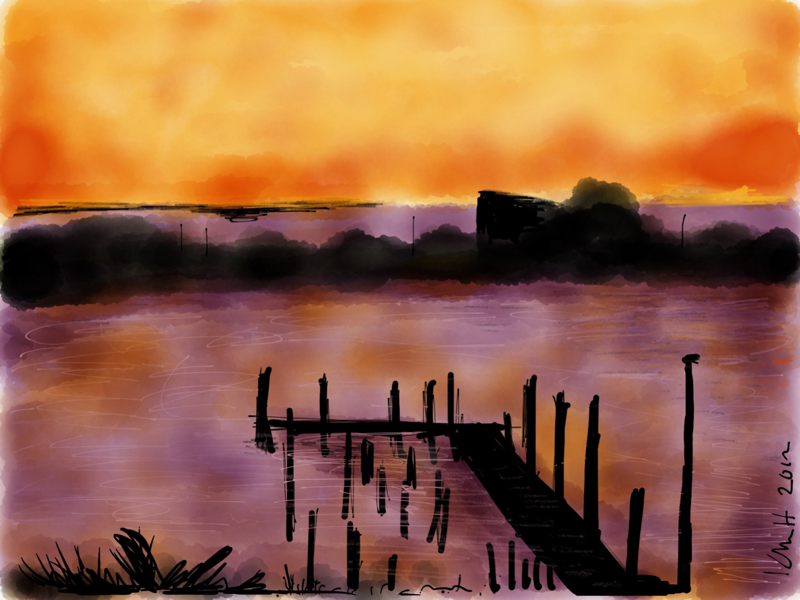This picturesque watercolor image, painted in striking hues of oranges, purples, and blacks, depicts a serene lakeside scene during either a sunrise or sunset. The upper quarter showcases a vibrant sky, blending soft yellow and bright orange shades, suggesting the sun's hidden presence. The lake below mirrors these warm colors, resulting in a mesmerizing interplay of purples and oranges across the water’s surface.

In the foreground, a somewhat dilapidated black dock extends from the bottom center, its weathered posts visible as they jut out from the water. To the left, black lines depict tall, graceful weeds, adding a touch of natural texture. Amongst these elements, subtle details such as small black dots near the horizon suggest distant islands or perhaps buildings and streetlights, their forms obscured by the radiant sky.

The artist's signature, partially legible with discernible letters "N," "H," and the year "2012," runs vertically along the right-hand side. This expertly crafted piece artfully combines a range of colors and details, presenting a beautiful and evocative snapshot of a tranquil waterside moment.